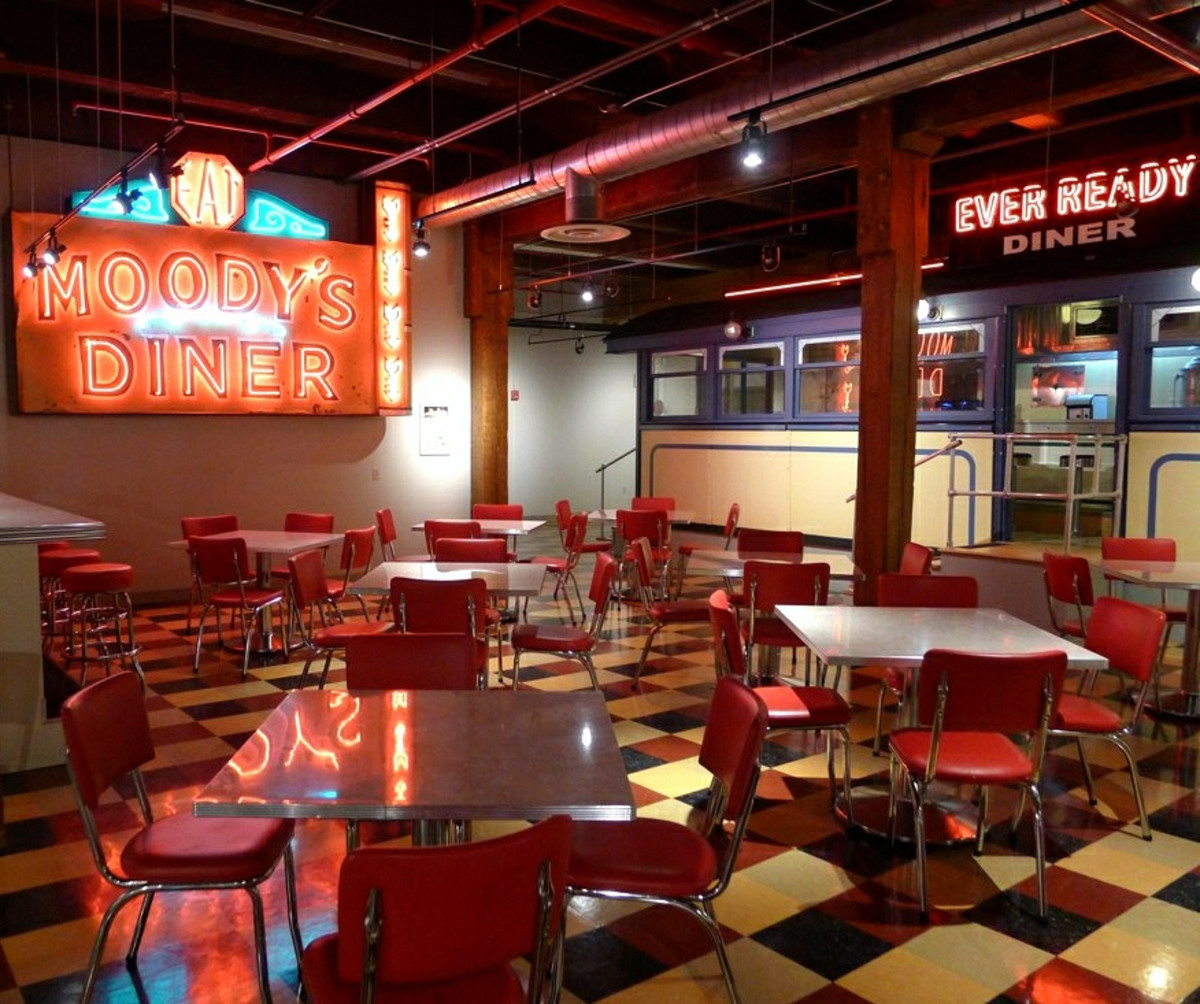This detailed photograph captures the inside of a quintessentially American diner, evoking a nostalgic 1950s atmosphere. The décor is dominated by a checkerboard floor composed of white, black, and vivid red squares. About ten metal tables with white tops dot the room, accompanied by standard red-cushioned metal chairs, each neatly arranged. 

At the top left corner of the image, a vibrant neon sign glows with the words "Moody's Diner," illuminated in dynamic orange, white, and blue hues. Above it, a smaller sign simply reads "eat." Adjacent to this, four vertically aligned mysterious figures, possibly depicting fish, capture your interest though their details remain a bit unclear.

To the top right, another striking neon sign reads "Ever Ready Diner," radiating a reddish-orange light. Below this sign lies what appears to be the entrance to the kitchen area. Complementing the vivid aesthetic, the walls are painted white, while the ceiling and pillars are accentuated in eye-catching red. Various exposed pipes crisscross near the ceiling, further enhancing the authentic, retro ambiance of the diner.